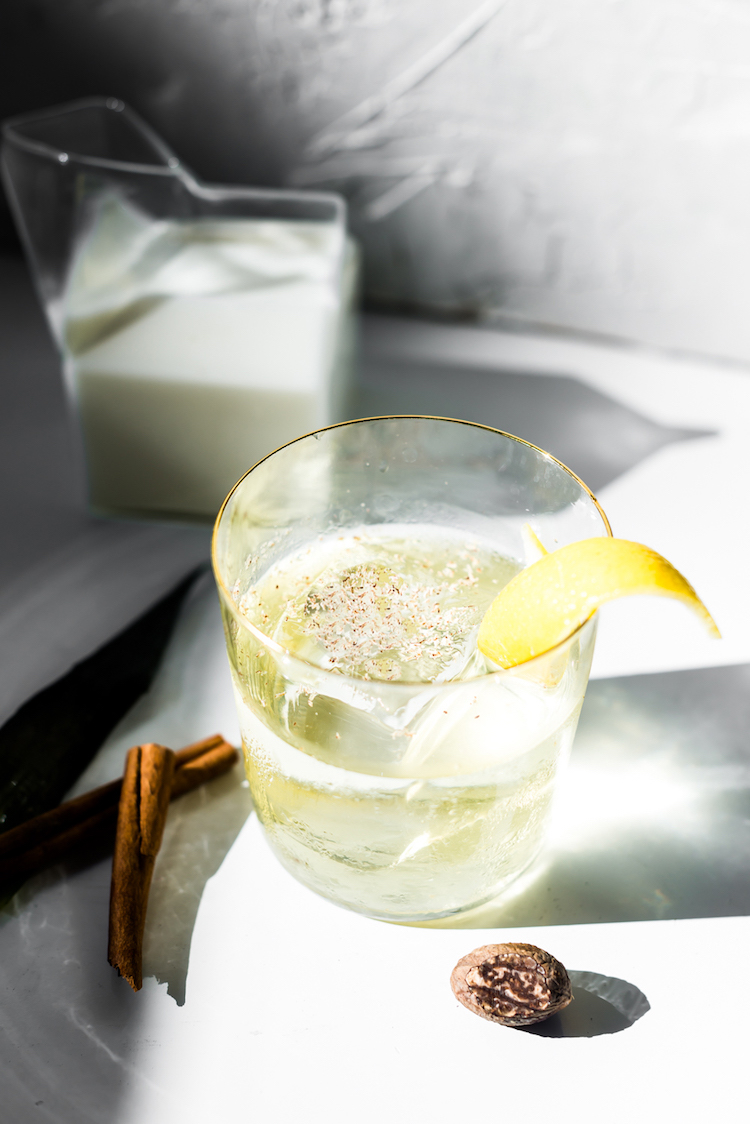This photograph features a close-up, sharply focused image of a fancy cocktail in a glass with a gold rim. The transparent golden drink has a lemon wedge adorning the rim and contains ice, with a sprinkling of what seems to be brown seasoning floating on the surface. At the base of the glass, on either side, are two cinnamon sticks and a nut, possibly a coffee bean. The setting is well lit, with light reflecting off the table surface. In the blurred background, there is a geometrically shaped glass or plastic container with a white liquid, likely milk or creamer. The entire scene, taken in portrait mode, boasts an aesthetic and sophisticated indoor environment with a predominantly white background and a clear chair visible in the top left corner.